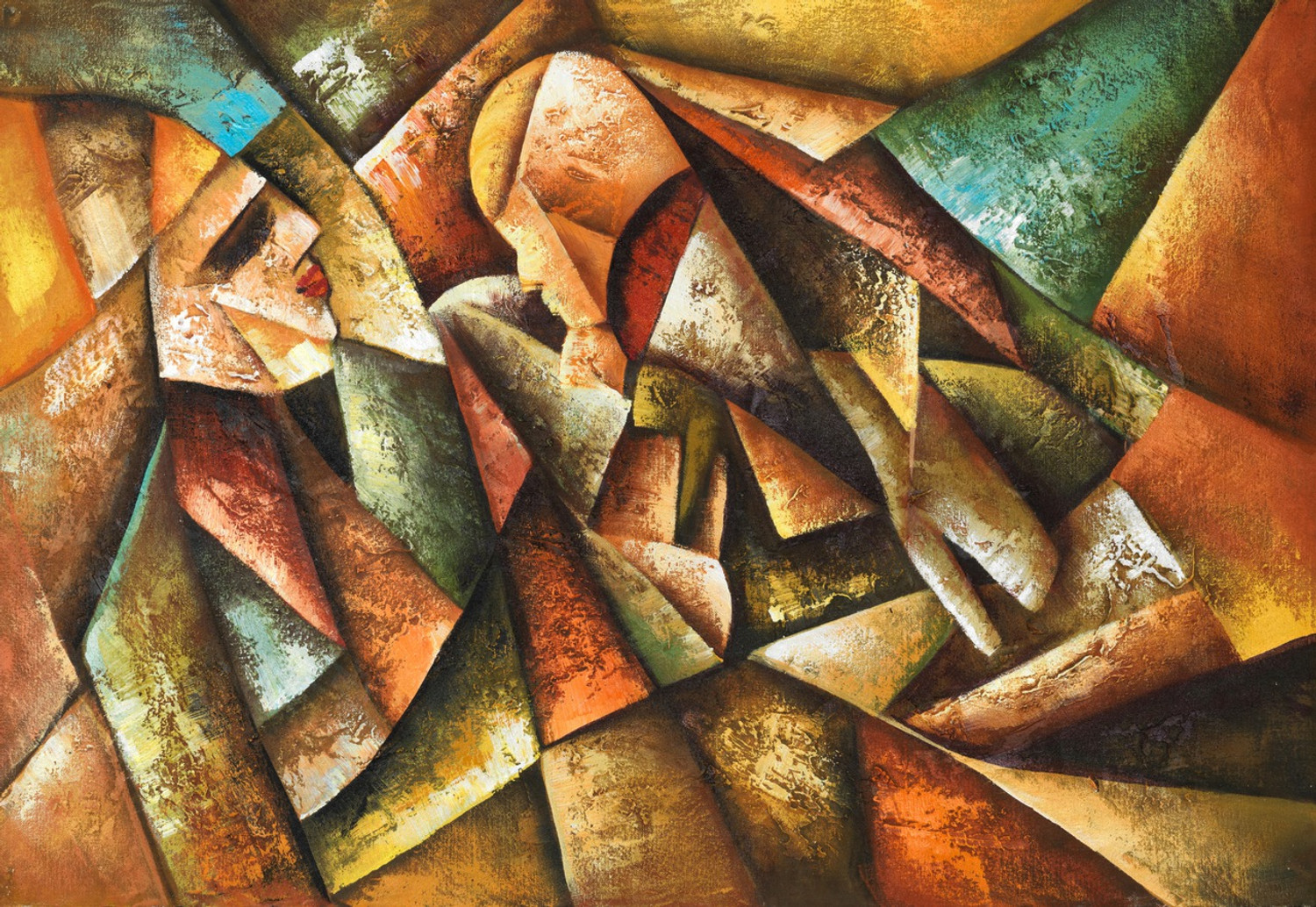The image is a highly abstract and impressionistic painting, primarily composed of a mosaic of triangular and geometric shapes with a textured, stone-like appearance. On the left side, the artwork features a woman's face with pink lips, black eyes, and a tan-orange complexion, accentuated by an orange neck and hat. Adjacent to her, towards the center, is a depiction of a child, characterized by yellowish hair, a tan face, and a neck shaded red and white.

The painting cleverly uses these angular shapes to not only define the mother and child but also to create a rich background of varied hues. In the upper left corner, there's a bluish-black shape, with surrounding areas featuring shades of yellow, brown, and green. The lower portions include an array of dark blue, white, red, and green shapes, adding to the painting's depth and complexity. The mother's arm is seen wrapped around the child, adding a touch of tenderness to the abstract composition. The overall impression is one of a sophisticated blend of abstract forms and impressionist elements, creating a visually compelling and emotionally resonant piece.